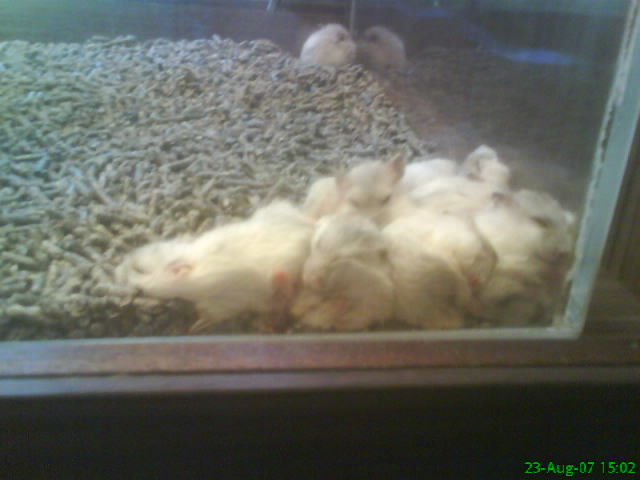A grainy close-up photograph, dated 23rd August 07 at 15:02, shows a glass terrarium or aquarium resting on a wooden table, potentially in a pet store or private home. Inside, the bedding consists of a substantial layer of small pellets, brown or black in color. Gathered in the lower right corner of the enclosure is a cluster of approximately 10 fluffy baby mice, predominantly white with some grey streaks, displaying little pink ears and feet. One solitary baby mouse is located in the upper right-hand corner, distinct from the huddled group. The overall quality of the image is low, making the details slightly blurred and the animals difficult to discern with complete certainty.